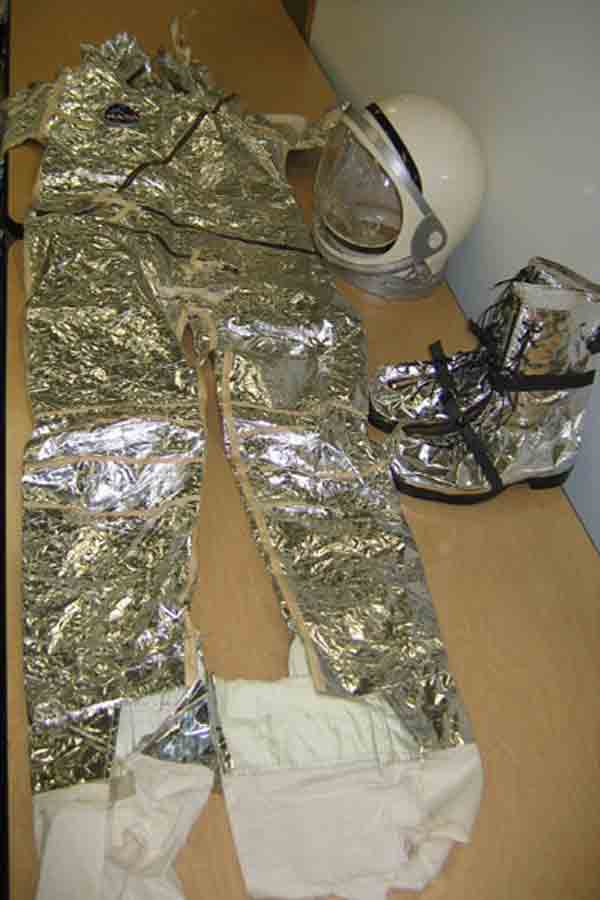In this detailed photograph, we observe a long, beige-colored table upon which an intricately crafted silver suit is displayed. The suit, reminiscent of a child's imaginative science project, appears to be made completely from shiny tin foil, designed to resemble either an astronaut suit or a stuntman outfit. The legs of the suit culminate in white sections that seem to accommodate boots or shoes. The torso, also constructed from tin foil, features a distinctive zigzag black line running horizontally across the waist. Positioned on the upper right side of the chest is a blue circular badge, presumably representing NASA, although the text is somewhat blurred.

Adjacent to the legs of the suit is a pair of matching shiny silver boots adorned with two black straps, with the toes oriented westward. Underneath the arm of the suit, a white helmet is neatly placed, intended for the astronaut to wear. The helmet is equipped with a clear shield, likely made of glass or plastic, designed to protect and provide visibility for the wearer.